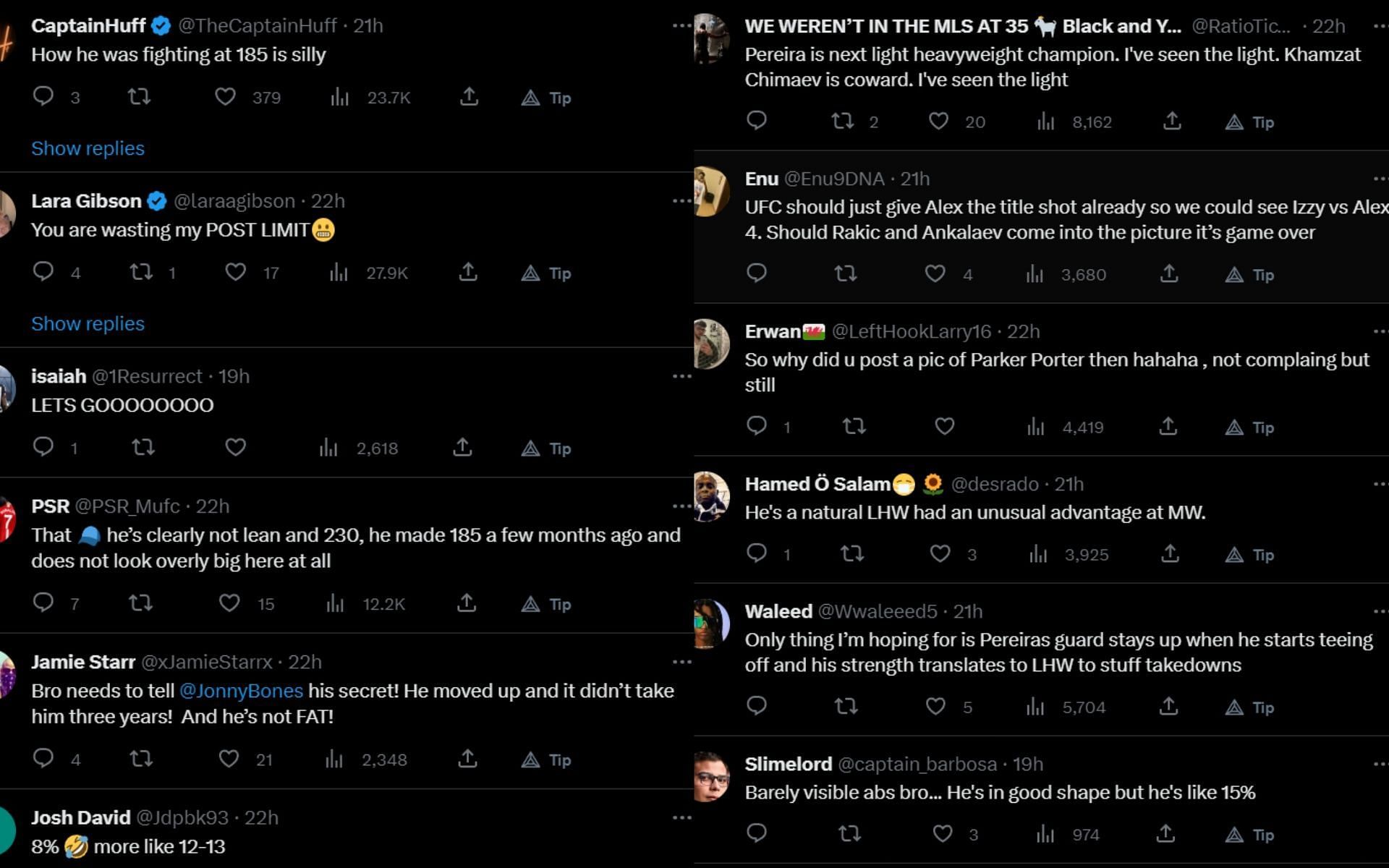The image is a screenshot captured within a mobile application, displaying a heated comment section. The interface features two columns of user comments against a black background with white text, creating a sharp visual contrast. 

**Left Column:**
At the top, there is a comment by a user named Captain Huff, critiquing someone's performance at 185 pounds. Below this, each comment has a series of icons indicating interaction metrics: a comments icon, a retweet icon, a heart icon with "379" likes, a views icon showing "23.7k" views, an upload icon, and a "tip" button.

Other contributors in the left column include Laura Gibson, who complains about wasting her post limit, and Isaiah, who enthusiastically exclaims, "Let's go" with multiple O’s. The thread continues with numerous other commenters such as Jamie Starr and ends with Joss David.

**Right Column:**
At the top right, it starts with a comment on not being in the MLS at 35, followed by a series of responses, echoing the structure of the left column and populated by various users, each accompanied by profile pictures—some realistic and others that appear to be avatars.

There are approximately 12 comments in each column, indicating a lively discussion with diverse participation.